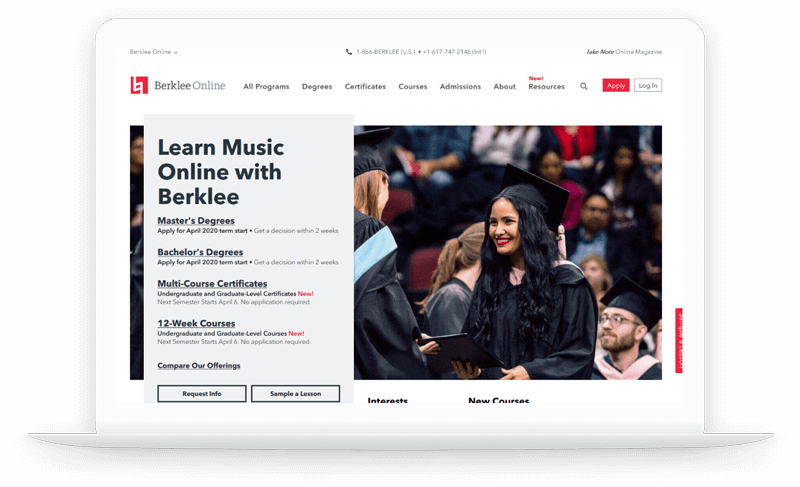In this image, we see a digital render of a sleek, white laptop displaying a webpage. The laptop appears pristine and modern, somewhat stylized, giving it a slightly artificial look. The screen is open to a website, specifically the homepage of Berklee Online. 

At the top of the page, there's a horizontal navigation bar. A drop-down menu is currently open, showing "Berklee Online." To the left of this menu, contact information is displayed, listing phone numbers: 1-866-BERKLEE for U.S. inquiries and 1-617-747-2146 for international inquiries. On the right side of the bar, there is a section titled "Take Note Online Magazine."

Below the navigation bar, the Berklee Online logo is prominently displayed—a red square with a stylized 'B' inside it. Adjacent to the logo are several categories: "All Programs," "Degrees," "Certificates," "Courses," "Admissions," "About," and "Resources." At the far right of this section, there's a magnifying glass icon for search functionality, a red "Apply" button, and a white "Log In" button.

Further down the page, there is a prominent photograph of a woman in a graduation cap and gown receiving a diploma from another woman. To the left of this image, the text reads: "Learn Music Online with Berklee." Below this heading, various academic offerings are listed: 

- "Master's Degrees: Apply for April 2020 Term Start"
- "Bachelor's Degrees: Apply for 2022 Term Start"
- "Multi-course Certificates: Undergraduate and Graduate Level Certificates"
- "12-week Courses: Undergraduate and Graduate Level Courses"

The overall layout is clean and structured, emphasizing Berklee Online's educational programs and easy navigation for prospective students.